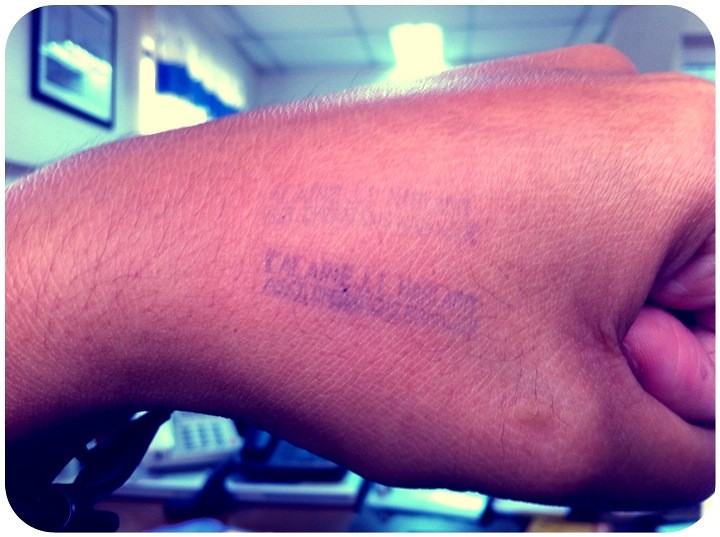In this detailed color photograph, presented in landscape orientation, the main focus is on a close-up of a man's left fist. The fist is extended from the left side towards the right, with part of the knuckles cut off on the right edge of the image. The thumb side of the hand is prominently visible, displaying a blue stamp that resembles a club or nightclub entry mark. The stamp features two lines of text: the upper line, which is faint and ghost-like, and the lower line, which reads "C-A-C-A-I-N-E, J period, T period" with parts of the text illegible. Additionally, there seems to be another unclear line beneath these two stamps. The background, suggesting an office or reception desk, includes elements such as overhead lighting, wall prints, windows with curtains, and a desk cluttered with items including telephones. Visible on the man's left hand is some arm hair and what looks like a mosquito bite at the base of the thumb, adding to the realism and detail of the scene.